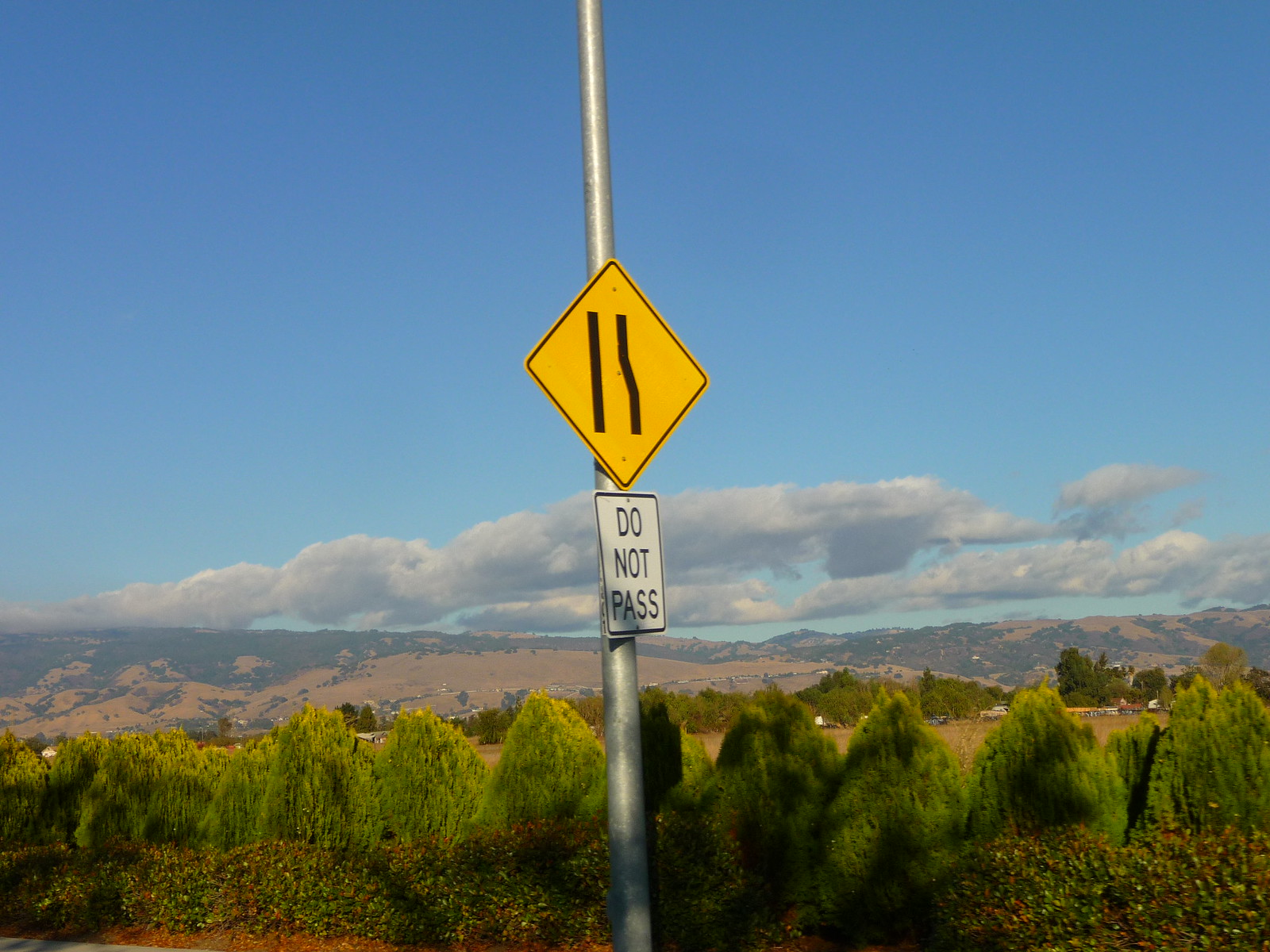This photograph, taken in a horizontal format, captures a captivating outdoor landscape. Dominating the foreground is a metal pole slightly off-center to the left, typically used for road signage. Attached to the pole is a yellow, diamond-shaped sign indicating the upcoming end of the right lane, with a white "Do Not Pass" sign positioned directly beneath it.

The midground features a mixture of gentle rolling hills and a dense line of trees, presenting a mosaic of earthy brown tones interspersed with patches of greenery. Though not lush, the vegetation adds a hint of verdancy to the otherwise arid terrain. Fields, varying in color and texture, stretch out between the viewer and the distant hills, creating a layered effect in the visual composition.

The upper half of the image is dominated by a flawlessly clear, vibrant blue sky, contrasting beautifully with the rugged landscape below. This expansive sky enhances the sense of depth and openness in the scene, making it a quintessential landscape photograph.

Overall, the image's detailed elements and harmonious balance between earth and sky create a visually pleasing and serene outdoor vista.